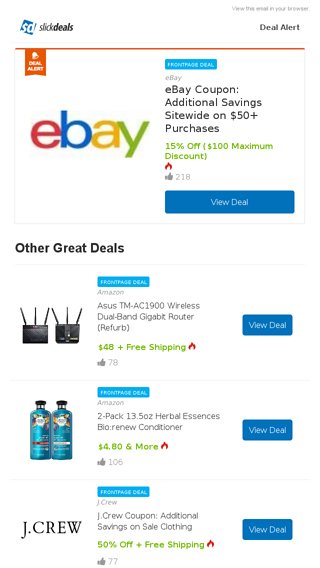This screenshot showcases a page from the eBay website featuring a selection of current deals. At the top-left corner, the page is headed by the "Slick Deals" logo with the initials "SD" beside it, adjacent to the "Deal Alert" label on the right. Faint, unreadable text sits above these elements. Centrally positioned is a prominent, multi-colored eBay logo—composed of red, blue, yellow, and green. Accompanying this is a heading "Important Deal," introducing an eBay promotion that offers a significant discount: an eBay coupon providing sitewide savings of 50% on purchases over $50, up to a maximum discount of $100. Beneath this announcement is a conspicuous "View Deal" button.

Below this primary promotion, the section titled "Other Great Deals" presents three featured items:

1. **Wireless Router**: An image displays two black routers under the headline "Front Page Deal Amazon." The specific product is the AsusTM-AC1900 Wireless Dual Band Gigabit Router (Refurbished) priced at $48 with free shipping. This deal has received a commendable 78 thumbs-up ratings. A "View Deal" button is available for further details.
   
2. **Herbal Essences Conditioner**: This includes a picture of the conditioner, advertising a 2-pack of 13.5 oz bottles of Herbal Essences Bio: Renew Conditioner listed at $4.80. The deal has garnered 106 thumbs-up ratings and a corresponding "View Deal" button.
   
3. **J.Crew**: Displayed as a simple text "J.Crew" in black, indicating a coupon offer. It highlights additional savings on sale clothing, offering a 50% discount plus free shipping. A "View Deal" button is provided.

This detailed screenshot offers a clear overview of promotional items, complete with descriptions, pricing, and user ratings.